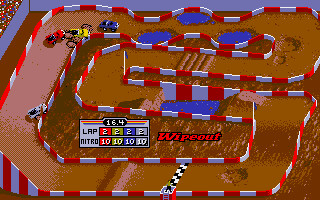The image is a screenshot from a video game featuring a dirt track with zigzagging paths and numerous obstacles, such as dirt hills and mud puddles. The track is delineated by a white and red-striped wall, extending along its perimeter. In the upper left corner, there are bleachers filled with an audience, adding to the competitive atmosphere. Prominently visible is a black and white finish line. Several monster trucks are mid-race, vying for position on the track. The screenshot includes a red "Wipeout" banner and a scoreboard displaying the number of laps and available nitro boosts for the players. The game seems reminiscent of titles like "Super Off Road" or "RC Pro-Am," where players control miniature vehicles and navigate intricate courses.